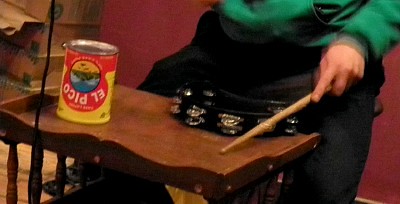In this image, we see a man sitting at a small, brown wooden table with decorative curves, reminiscent of vintage furniture. He is wearing a green sweatshirt with a central pocket and black pants, sitting on a stool, with his face out of the frame. The man holds a single tan drumstick in his left hand, tapping it on the table near a black and silver tambourine. On the far left side of the table lies an upside-down red and yellow can labeled "El Pico," possibly used as a percussion surface. A black cord hangs down on the left side, and boxes are piled on the floor in the background. The wall behind him is a dark, almost maroon red.